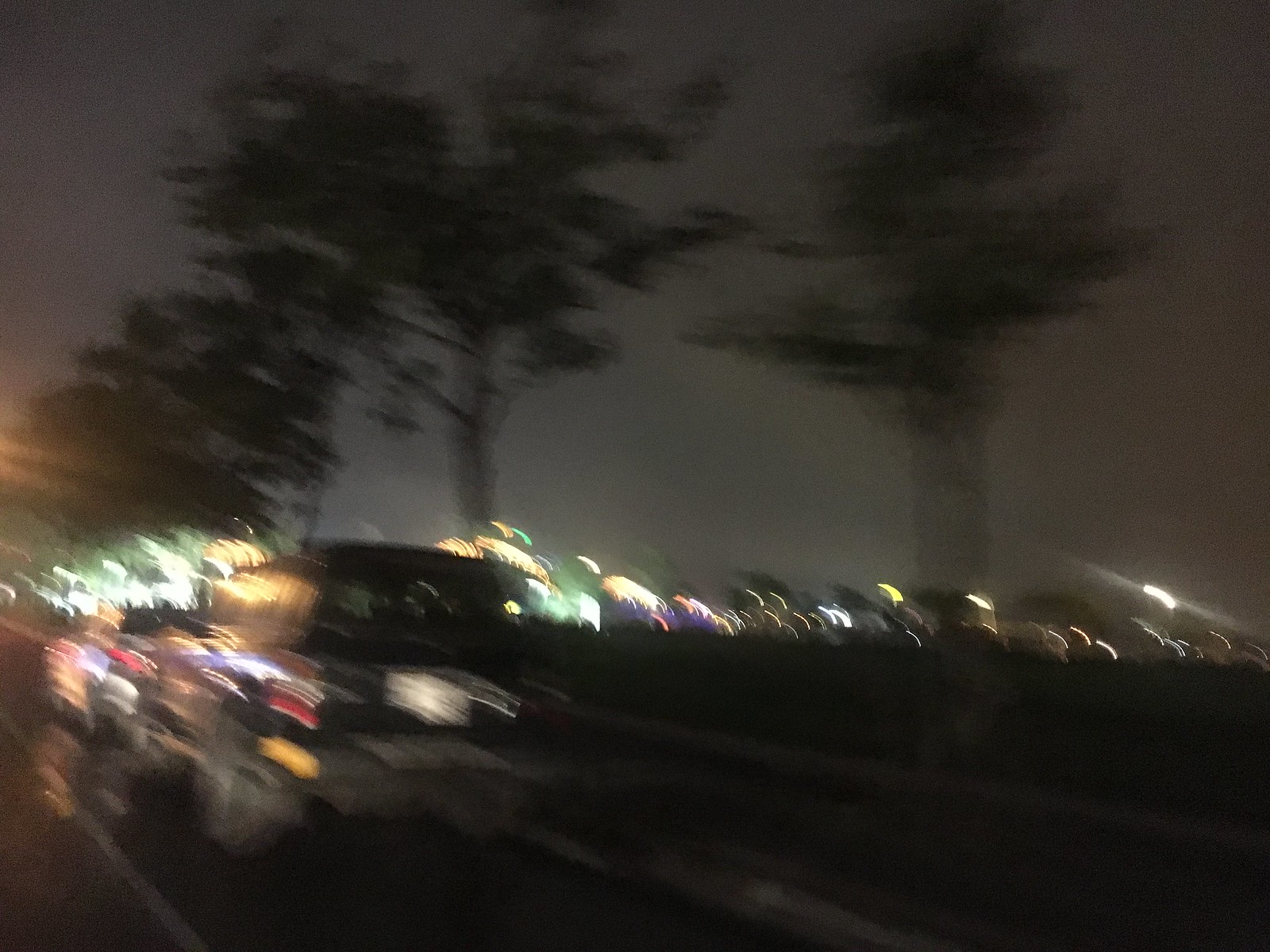A nighttime scene captures a road glistening under possible recent rainfall, with visible white lane markings. Two cars dominate the frame—a dark SUV closely following a silver sedan. Both vehicles have their taillights illuminated, and the blurry glow of the license plate lights adds to the scene's mystique. Towering trees with lengthy trunks and leafy canopies line the roadside. In the distance, an open field stretches out, peppered with a multitude of colorful lights, hinting at a carnival or some other vibrant attraction, though the image's heavy blur leaves the details indistinct.